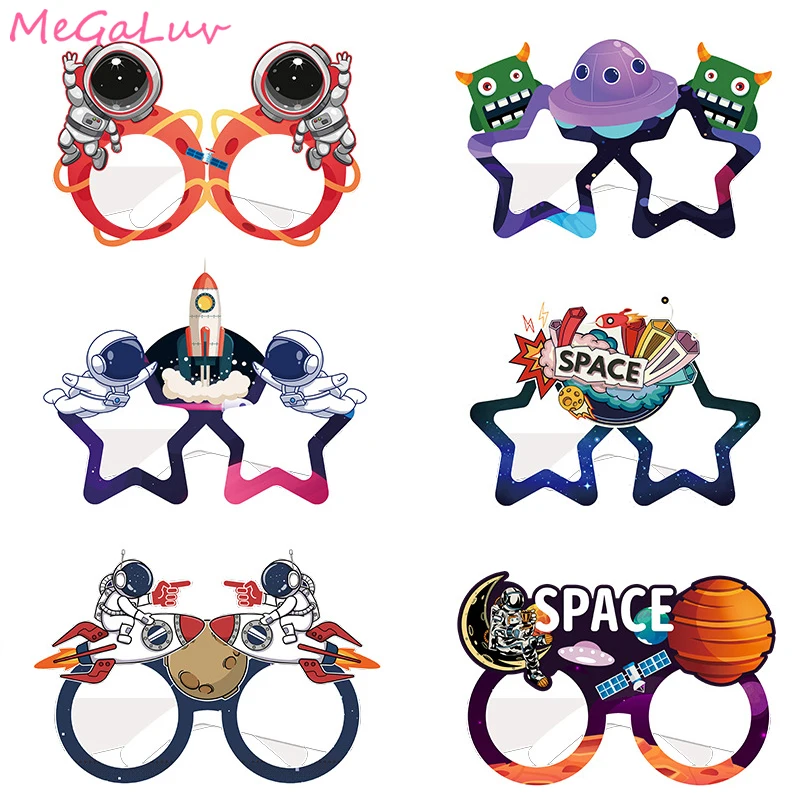The image features six uniquely designed glasses, each with a space-themed motif, arranged in two rows against a white background. In the top left, a pink cursive text reads "Me Ga Love" above a pair of red glasses adorned with two astronauts in white suits and black helmets, seemingly greeting with outstretched arms. To the right, another pair of glasses shaped like stars showcases two green aliens with yellow horns and red eyes, with a purple UFO in the center. Continuing in the top row, a blue and pink star-shaped pair of glasses displays an astronaut and starry design set against dark blue.

In the bottom row, the far left features blue oval glasses with two astronauts positioned on red and white rockets, mimicking a pointing gesture, with the slogan “SPACE” underneath. Next, there is a star-shaped pair displaying the word “space” alongside colorful details like a small rocket and crescent moon. Finally, to the far right, purple oval glasses exhibit an orange planet (resembling Mars) on the right, a black moon with an astronaut perched on it in the center, and a blue and white satellite to the left.

Combining colors and motifs, each pair depicts different adventures from space, featuring astronauts, aliens, rockets, and celestial bodies, all laid out in an imaginative and vibrant design.